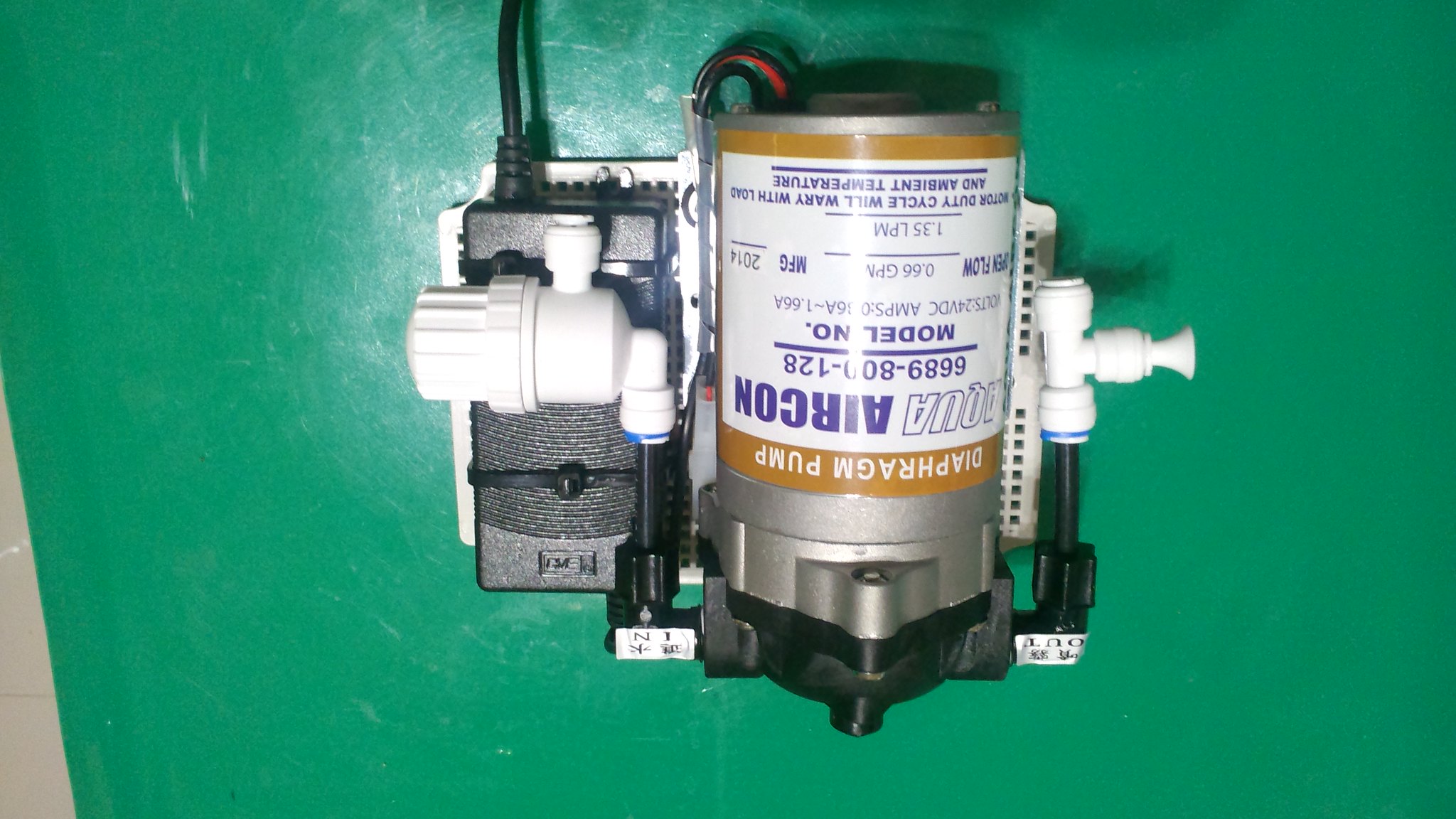The image features a small mechanical device known as a diaphragm pump, shown with an upside-down perspective against a solid green background. The pump, comprising a metal cylinder, has red and black wires extending from what appears to be the bottom, but is actually the top due to the flipped orientation. These wires indicate the pump is plugged into an outlet. The cylinder is adorned with a label that has a tan stripe and white background. "Diaphragm Pump" is written in white font within the tan stripe, whereas "Aqua Aircon 6689-80(9 or 0)-128" is inscribed below in blue letters on the white part of the label. This label also mentions specifications about the amperage (amps), flow rate in liters per minute (LPM), and notes that the duty cycle varies with load and ambient temperature. Additionally, the pump has black plastic components screwed onto its metal body and plastic pipes extending from it.